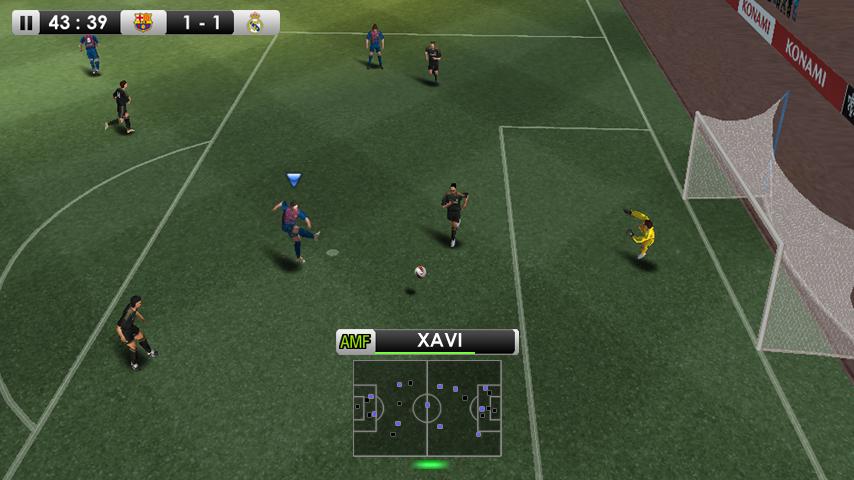Screenshot from a Konami Video Game: Barcelona vs. Real Madrid Football Match

In this detailed screenshot from a Konami-produced football video game, a match between FC Barcelona and Real Madrid is in progress, as indicated by the team logos prominently displayed in the top left corner. The game clock reads 43 minutes and 39 seconds. The screen shows a pivotal moment with a Barcelona player, identified as Xavi (AMF), poised to take a shot towards the goal. His player icon is highlighted on a mini-map of the field, which features little purple blocks and a small green light.

The Barcelona player is easily identifiable by his team's iconic kit, while the goalkeeper from Real Madrid is clad in a distinctive yellow uniform. Bunting in the background displays the Konami logo, both in white on a red rectangle and in red on a white rectangle, clearly marking this game as a product of Konami. Despite the vivid details, the exact title of the football game remains unspecified.